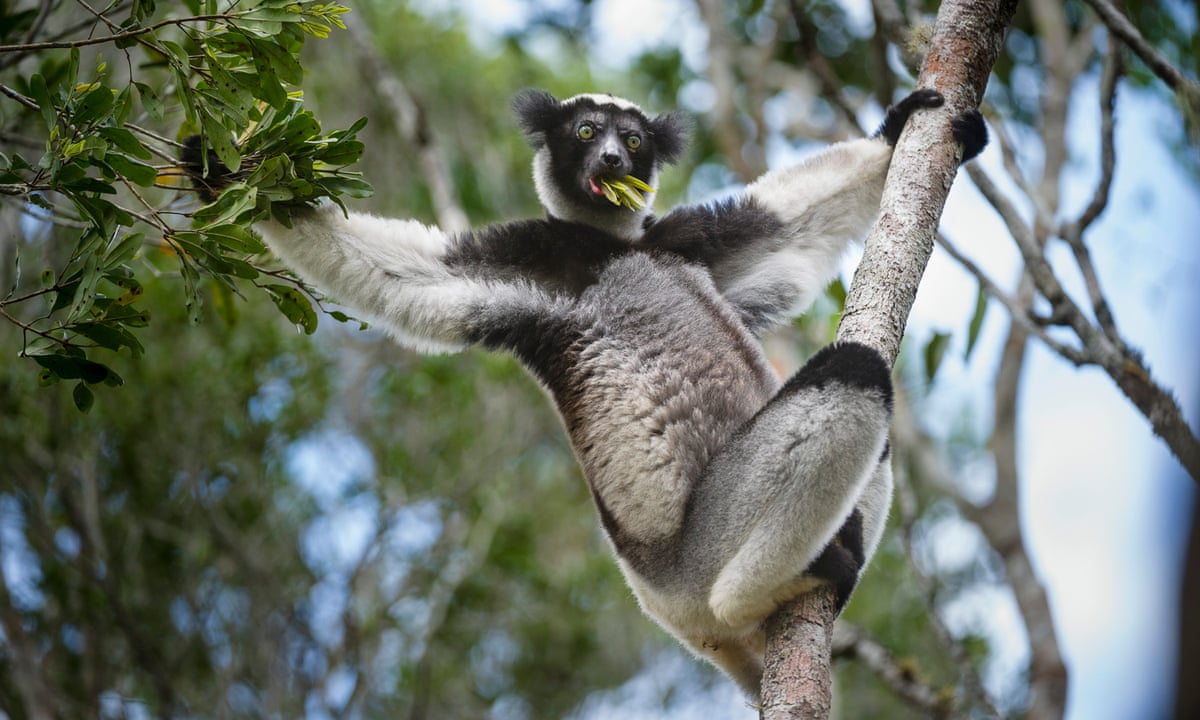The image features a black and white lemur perched on a thin, branchless tree trunk with a few leaves in its mouth. The lemur, which has very fluffy and furry white fur on its belly and arms, and black fur on its knees and shoulders, is grasping the tree trunk with its left hand while its right hand is extended towards another tree, holding onto a branch. It has large, round green eyes and two big ears protruding from the sides of its head, reminiscent of Mickey Mouse. Both of its feet are wrapped around the trunk, and the tail is visible, hanging down and slightly obscured behind the trunk. The background includes additional trees and branches, with a clear blue area that could be the sky on the far right. The lemur appears to be intently staring ahead as it munches on the leaves.